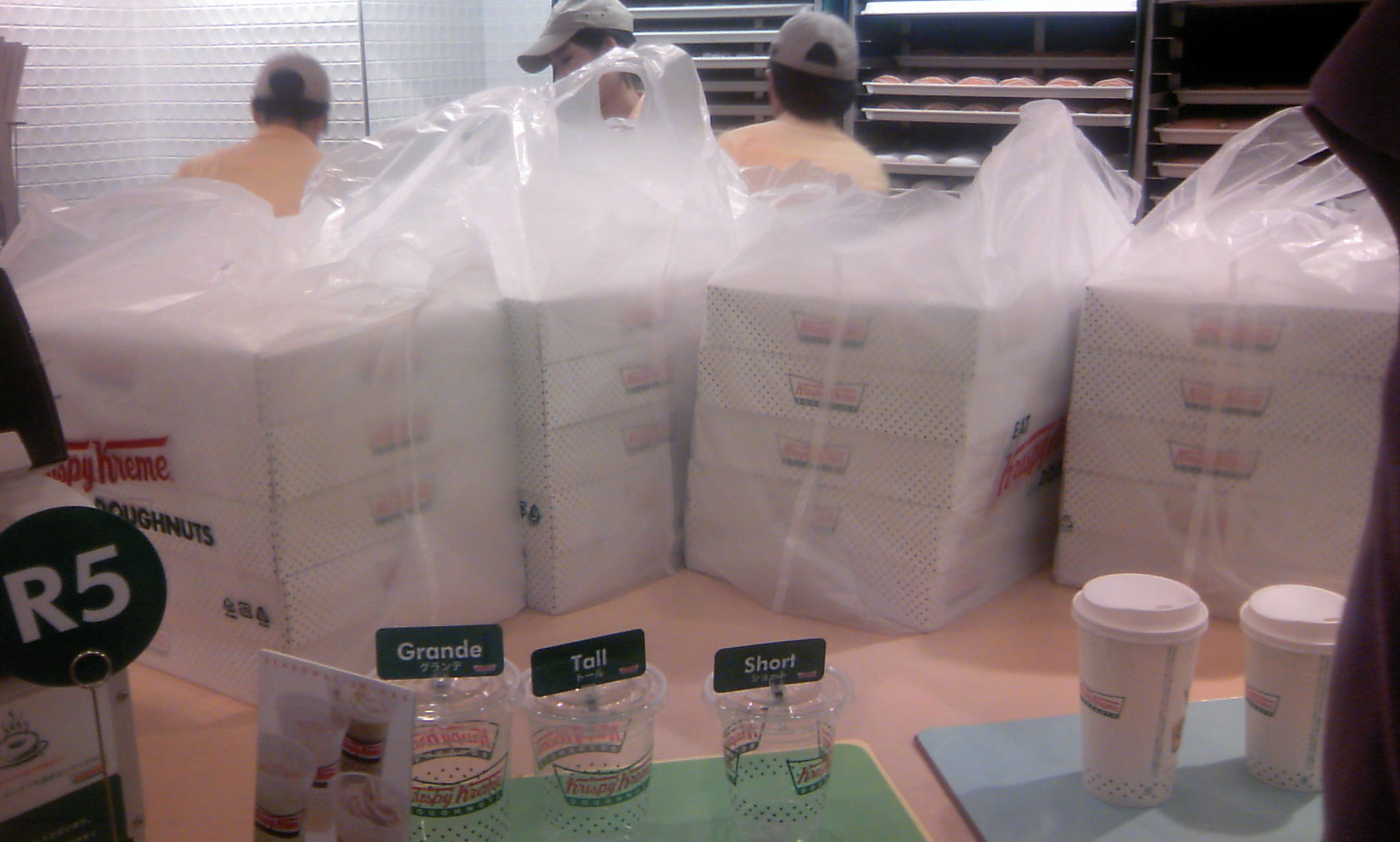The color photograph captures the interior of a vibrant Krispy Kreme store. In the foreground, arranged on a table, are four clear plastic tote bags, each containing five boxes of Krispy Kreme donuts stacked neatly. The boxes prominently display the Krispy Kreme logo. In front of these bags, there is a lineup of clear plastic drink cups labeled Grande, Tall, and Short, each bearing the Krispy Kreme branding. Adjacent to these, on green and blue placemats, are several insulated paper cups with white sippy lids designated for hot beverages.

In the bottom left corner of the image, a chrome sign holder with a circular sign marked "R5" stands out. Moving to the background, three employees are visible, all wearing tan baseball caps and light orange shirts. The workers are busy behind the glass counter, though they are partially obscured by the tote bags in the foreground. The central worker is seen in profile, while the others are shown from the back. Tall metal proofing racks filled with trays of baked goods, likely fresh donuts, stand behind them, adding to the bustling atmosphere of the store.